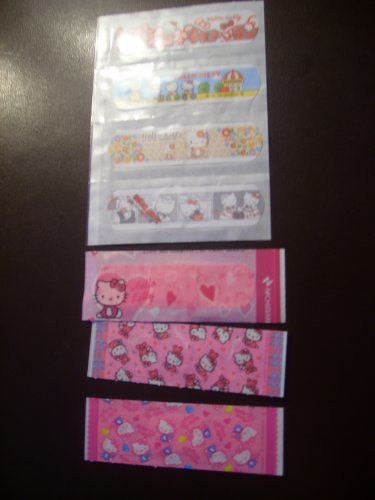This color photograph, oriented in portrait mode, captures a neatly arranged collection of children's band-aid wrappers displayed on a black background, possibly a table or paper. The image features a total of seven unopened band-aid packages, each showcasing vibrant and detailed designs. The top four band-aid wrappers are colorful and individually wrapped in white packaging, featuring a variety of playful patterns including the iconic Hello Kitty design. Below them are three larger band-aid wrappers, uniformly styled with a pink background adorned with the Hello Kitty logo and red hearts. The bottom three wrappers slightly overlap one another, with the bottom package lying flat and fully visible. The overall composition is crisp and clean, exemplifying the style of product photography with a focus on realism and representationalism.